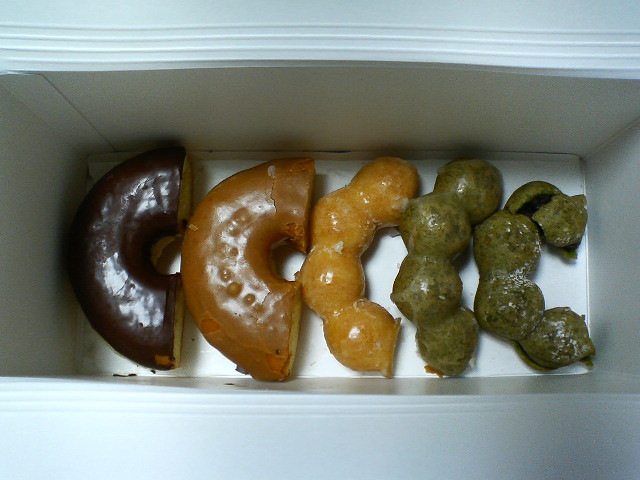This photograph, taken from above, showcases a white rectangular cardboard box containing five meticulously cut donut halves, placed on a white table. From left to right, the first donut half is chocolate glazed, featuring a rich dark brown coating. The second donut half appears to be pumpkin spice with a light brown glaze. The third is a unique donut composed of four interconnected, bead-like segments, coated in a plain glaze. The fourth and fifth halves are similar to the third, but they are covered in a distinct dark green glaze, suggesting a possible pistachio flavor. Notably, one of the green-segmented donut halves has a damaged segment, slightly detached from the rest. The box fits the donut halves perfectly, and there are no crumbs beneath them, highlighting the precision with which they were cut, likely with a very sharp knife.